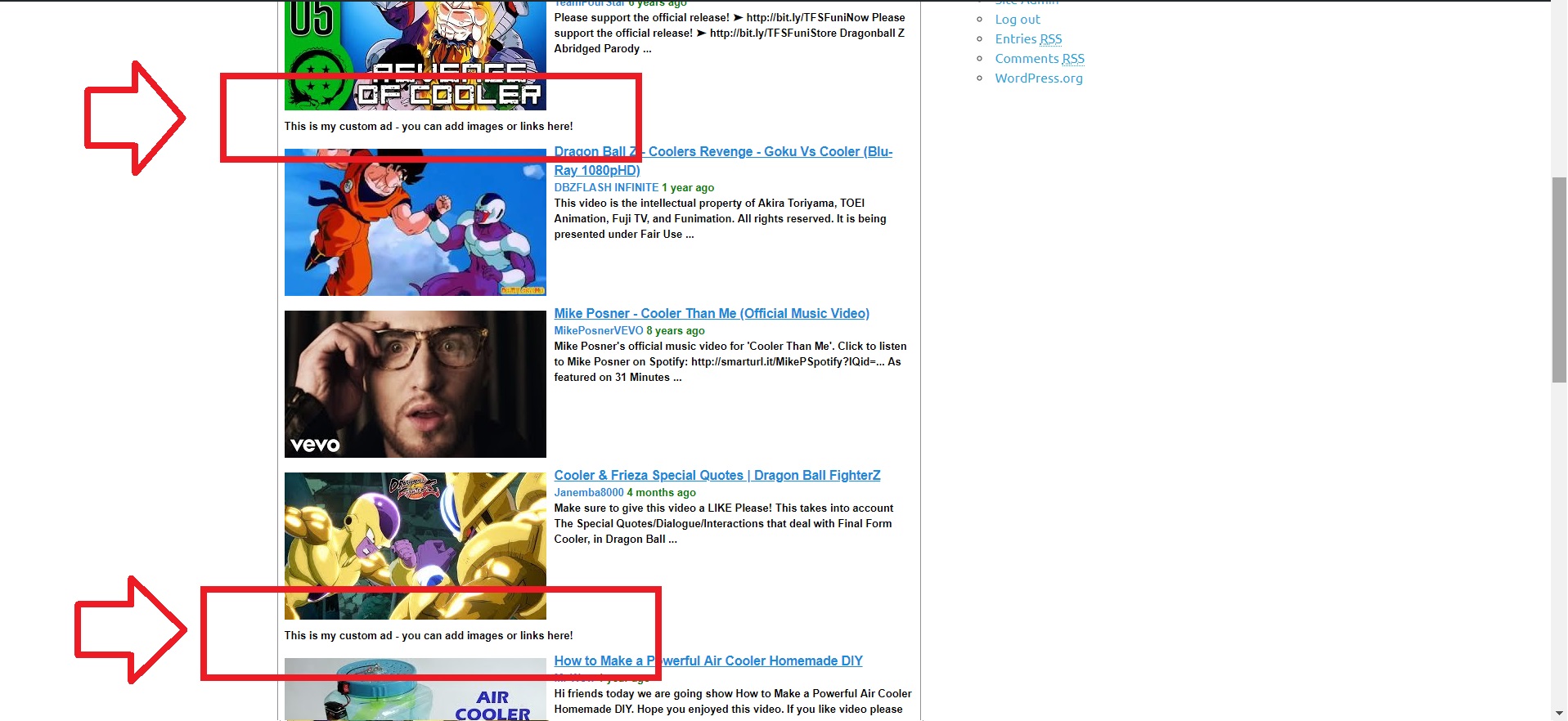This is a screenshot from a website interface. The background is predominantly white. Across the top, there is a thin black border. Down the left side and partially down the right side, about an inch wide, runs a very light grayish-blue border. Overlaying this on the left side is a darker gray stripe, about an inch down from the top.

Approximately an inch from the top on the left side, there is the outline of a red arrow pointing to the right. Adjacent to the arrow is a red rectangular outline, which overlaps two different videos.

The top video within this red rectangle features a thumbnail with a green border. The text reads "Revenge" at the top, "Cooler" beneath it, and within the red rectangle, it says: "This is my custom ad. You can add images or links here." To the right of this thumbnail is additional information about the video.

Below this, another video thumbnail displays a blue sky and a man in an orange shirt descending diagonally from the left, appearing to punch another man in front of him. The man being punched has black hair and wears a purple and gray suit. To the right of this thumbnail, there is more information about this video.

Underneath this, there's a close-up picture of a man's face with black-rimmed glasses, eyes wide open, mouth slightly ajar, and a goatee, looking straight at the camera. His hand is raised to his glasses. The logo "VEVO" is visible in the bottom left corner of this image, and to the right is additional information about this video.

The next video shows a yellow robot with a purple head and mouth area on the left side, running towards a red metal robot on the right. Detailed information about this video is presented to the right of the thumbnail.

This section is again overlapped by a red rectangular outline similar to the one above, with a red arrow pointing right next to it. Inside this rectangle, the text reads: "This is my custom ad. You can add images or links here."

The last, partially visible video at the bottom displays a blue background and the top part of a clear plastic container with a plastic lid. It features the text "Air Cooler" in purple. Information about this video appears to the right.'